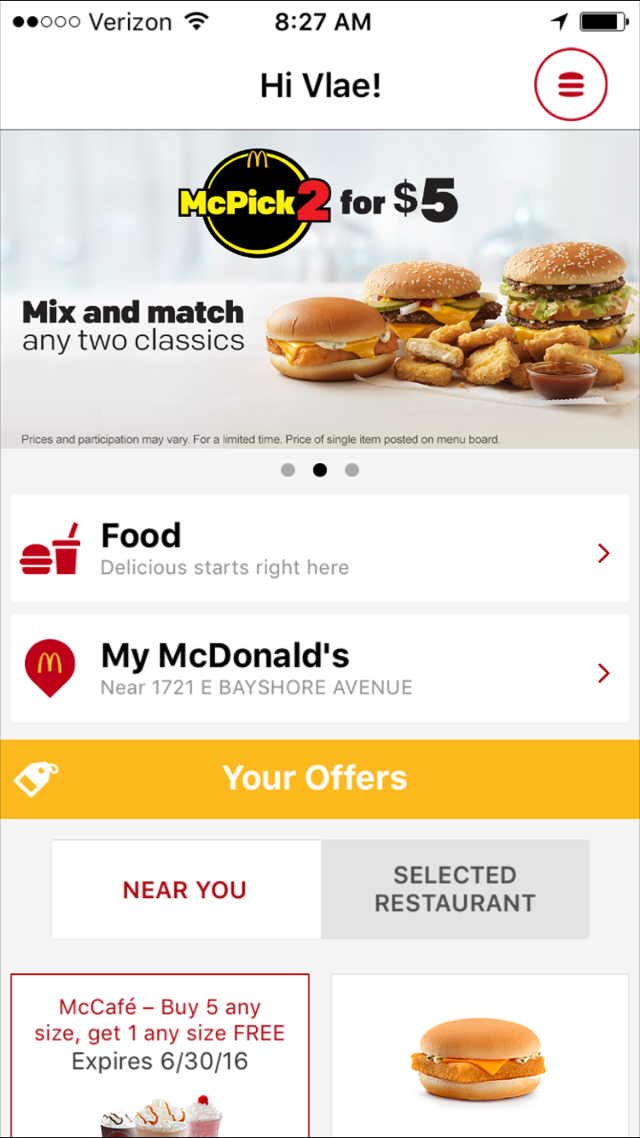Screenshot of the McDonald's App on a Smartphone

The image captures a screenshot from a smartphone displaying the McDonald's app interface. Ensuring all pertinent details are included, the top left corner of the screen shows the carrier name, "Verizon," along with icons for Wi-Fi, signal coverage, and the time, 8:27 AM. The battery icon, mostly full, is visible on the right.

In the main content area of the app, a greeting is displayed: "Hi Vlae," with the user's name in capital letters. Below the greeting, there’s a photograph of popular McDonald's menu items: a Filet-O-Fish sandwich, two hamburgers, and a generous pile of Chicken McNuggets accompanied by a small plastic container of dipping sauce.

Prominent text declares, "McPick 2 for $5. Mix and match any two classics. Prices and participation may vary. Offer valid for a limited time. Price of single item posted on menu board." Following this, a section titled "Food" bears the slogan "Delicious starts right here," accompanied by red illustrations of a burger and a soft drink.

The "My McDonald's" section uses a location pin marked with the iconic McDonald's golden arches to indicate a selected restaurant near "1724 E. Bayshore Avenue." The segment "Your offers" displays available deals: "Near you" and "Selected restaurant." Among the offers is a promotion for McCafé beverages: "Buy five any size. Get one any size free. Expires 6-30-16."

Lastly, the bottom of the screen features a photograph of three milkshake-type drinks, followed to the right by a partially visible image of a Filet-O-Fish sandwich, cut off at the bottom with no accompanying text.

This ornate screenshot exemplifies the functional and promotional elements of the McDonald's app, designed to enhance user engagement through personalized greetings, enticing visuals, and limited-time offers.